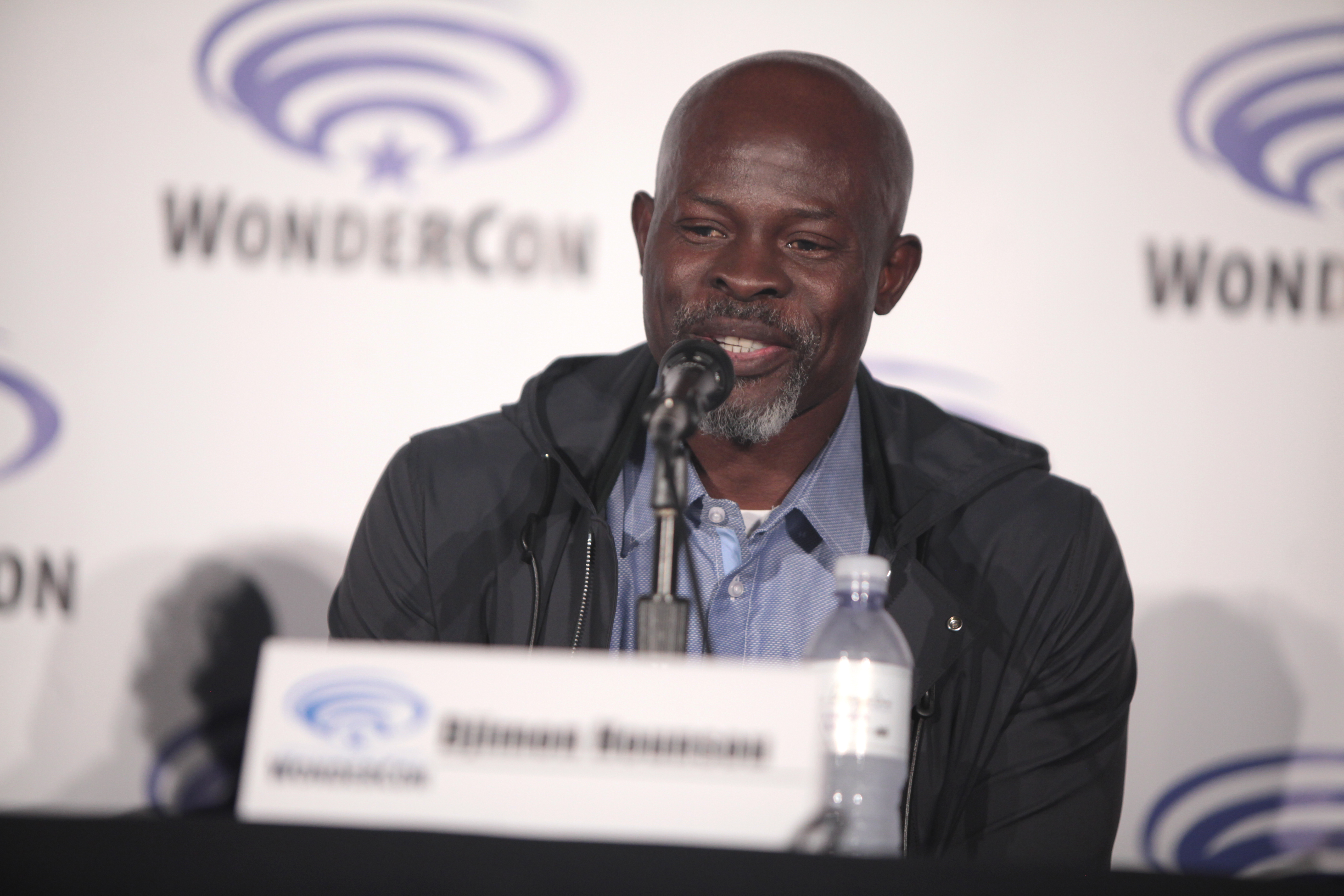In the image, a middle-aged, dark-skinned, bald man is seen speaking into a microphone at a podium, likely participating in a panel or Q&A session at WonderCon, as indicated by the repeated "WonderCon" branding in purple behind him. The background features a stylized design consisting of concentric purple swirls with a star at the center. The man is dressed in a dark gray jacket with a hood, a blue shirt with an open collar, and a white t-shirt underneath. He has a light mustache and beard, slightly graying at the edges. In front of him, there's a blurred name placard and a plastic water bottle with the cap still on.